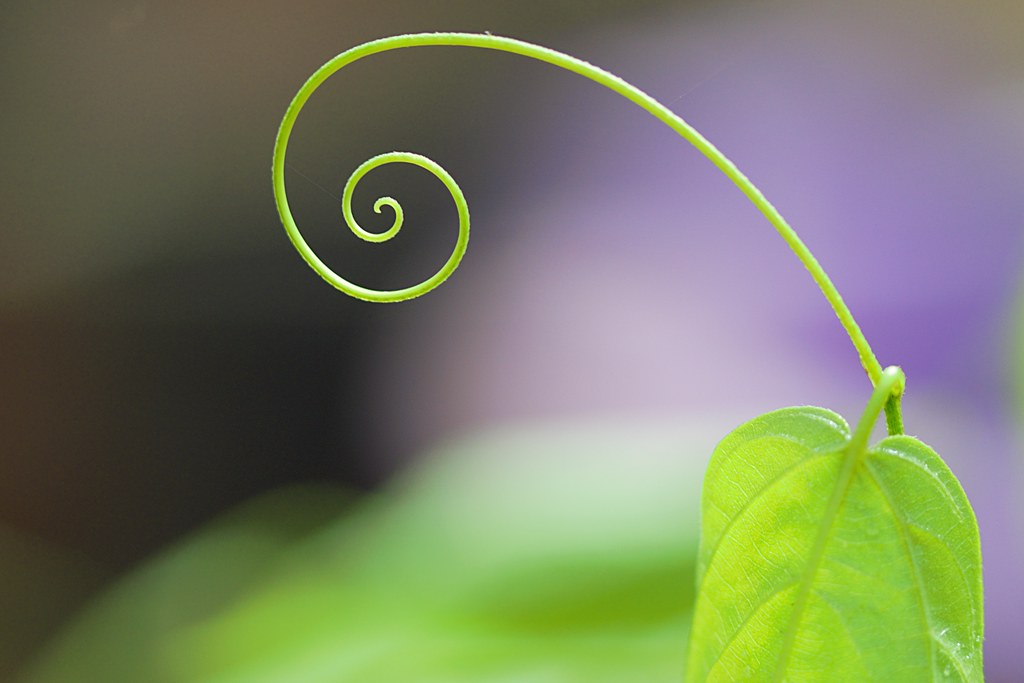This close-up image captures a vibrant, bright yellow-green leaf and its delicately curling stem, which forms a snail-shaped curve. The focal points are vivid and sharp, showcasing the intricate veins of the leaf and the elegant twist of the stem. The stem starts from the bottom-right of the image and extends upwards toward the center before curling at the end. The background is thoroughly blurred, with a mix of purples and greens, and transitions into dark and grayish-tan hues at the upper left, making the leaf and stem stand out prominently. The colors suggest the leaf is bathed in sunlight, enhancing its vivid and lively appearance. This detailed and artistic photograph likely serves an illustrative purpose, potentially for an identification manual for leaves.